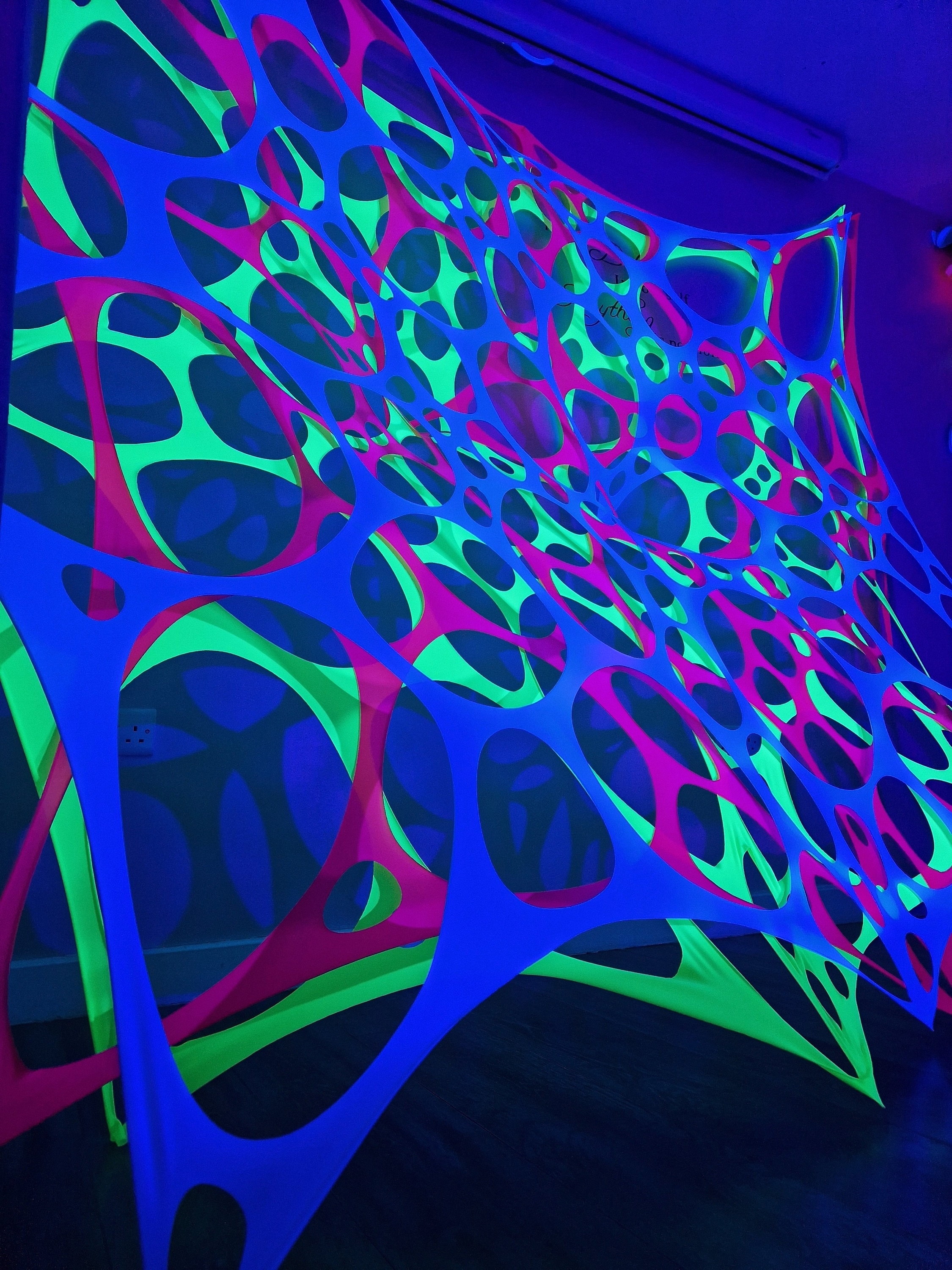This image captures an intricate art installation bathed in dark blue neon lighting. The room, featuring a ceiling and floor both tinted in various shades of blue, creates a captivating atmosphere that hints at either an art exhibit or a blacklight event. Dominating the wall and cascading towards the floor is a mesmerizing array of multi-colored, plastic-like webbing. This includes overlapping layers of stretchy fabrics adorned with irregular, large circular cutouts. The first layer at the back is a glowing lime green tarp, followed by a bright fuchsia, and topped with a dark blue web-like structure. Each layer has unique cutouts that do not perfectly align, contributing to a dynamic 3D effect. The rich colors of lime green, magenta pink, and royal blue are accentuated by the blacklight, giving the installation a vivid, fluorescent glow. The overall effect is a striking blend of color, light, and texture that transforms the room into an immersive neon spectacle.